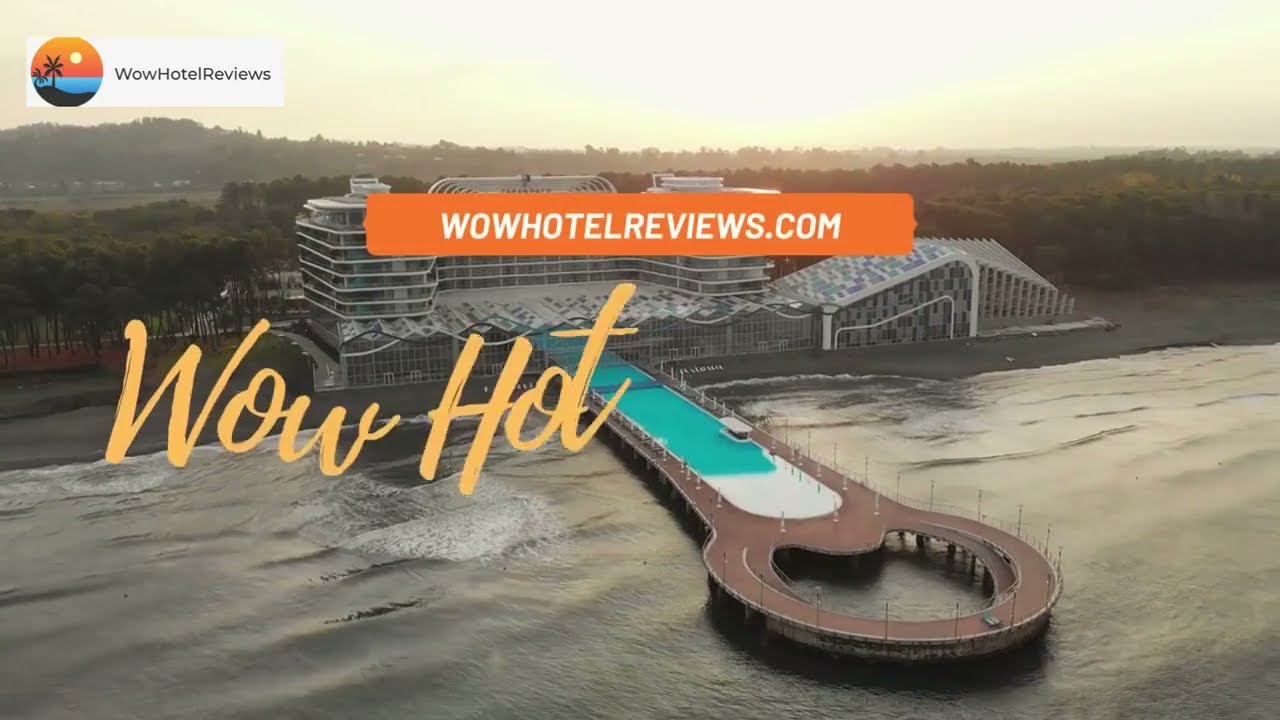This vibrant aerial photograph, featured as part of an advertisement for the website WowHotelReviews.com, captures a sprawling beachside hotel bathed in the warm hues of a setting sun. From its prominent position at the water’s edge, the hotel boasts a unique running track that encircles a vast central swimming pool, extending out towards the clear, shimmering ocean. The expansive complex includes a towering six-story building with a possible rooftop restaurant, offering breath-taking views of the horizon. 

On the upper left corner of the image, you can see the logo of Wow Hotel Reviews—a stylized sunset over an ocean backdrop framed by palm trees. Below it, the website's name, "WowHotelReviews.com," stands out in bold white letters within an orange stripe. The phrase "Wow Hot" is also prominently displayed in flowing yellow text in the middle left of the photograph. The lush green trees lining the shore enhance the resort's allure, underscoring the luxurious escape it promises. The ad implies that through WowHotelReviews.com, travelers can discover such magnificent accommodations at the best prices, ensuring a luxurious beachside stay.